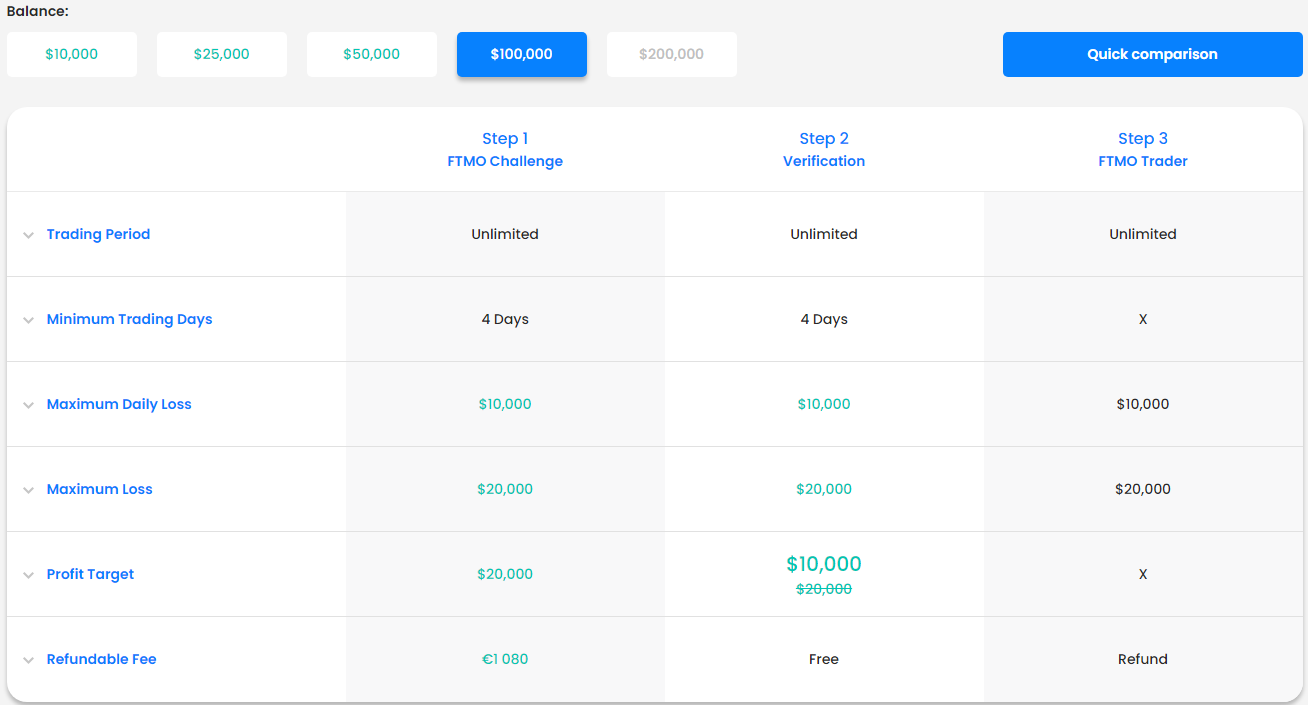The image is rectangular, slightly wider than it is tall, and features a gray background at the top. In the very top left corner, the word "Balance" is prominently displayed in bold print. Below this are five tabs with different monetary values: $10,000, $25,000, $50,000, $100,000, and $200,000. The $100,000 tab is highlighted with a blue background.

In the top right corner of the image, a blue button labeled "Quick Comparison" is visible. Below this top section, the layout transitions into a table format with several columns and rows. The columns are labeled Step 1: FTMO Challenge, Step 2: Verification, and Step 3: FTMO Trader.

On the left side of the table are various metrics: Trading Period, Minimum Trading Days, Maximum Daily Loss, Maximum Loss, Profit Target, and Refundable Fee. These are followed by corresponding entries under each step. For Trading Period, the entry is "Unlimited" for all three steps. The Minimum Trading Days row doesn't seem to have a specified entry.

The Maximum Daily Loss is listed as $10,000 under each step. For the Profit Target, Step 1 shows $20,000, while Step 2 has $20,000 crossed out and replaced with $10,000. For Step 3, there is an "X" marked in the row. Lastly, under Refundable Fee, for Step 1, it is listed as EUR 1,080, for Step 2, it is marked as "Free," and for Step 3, it states "Refund."